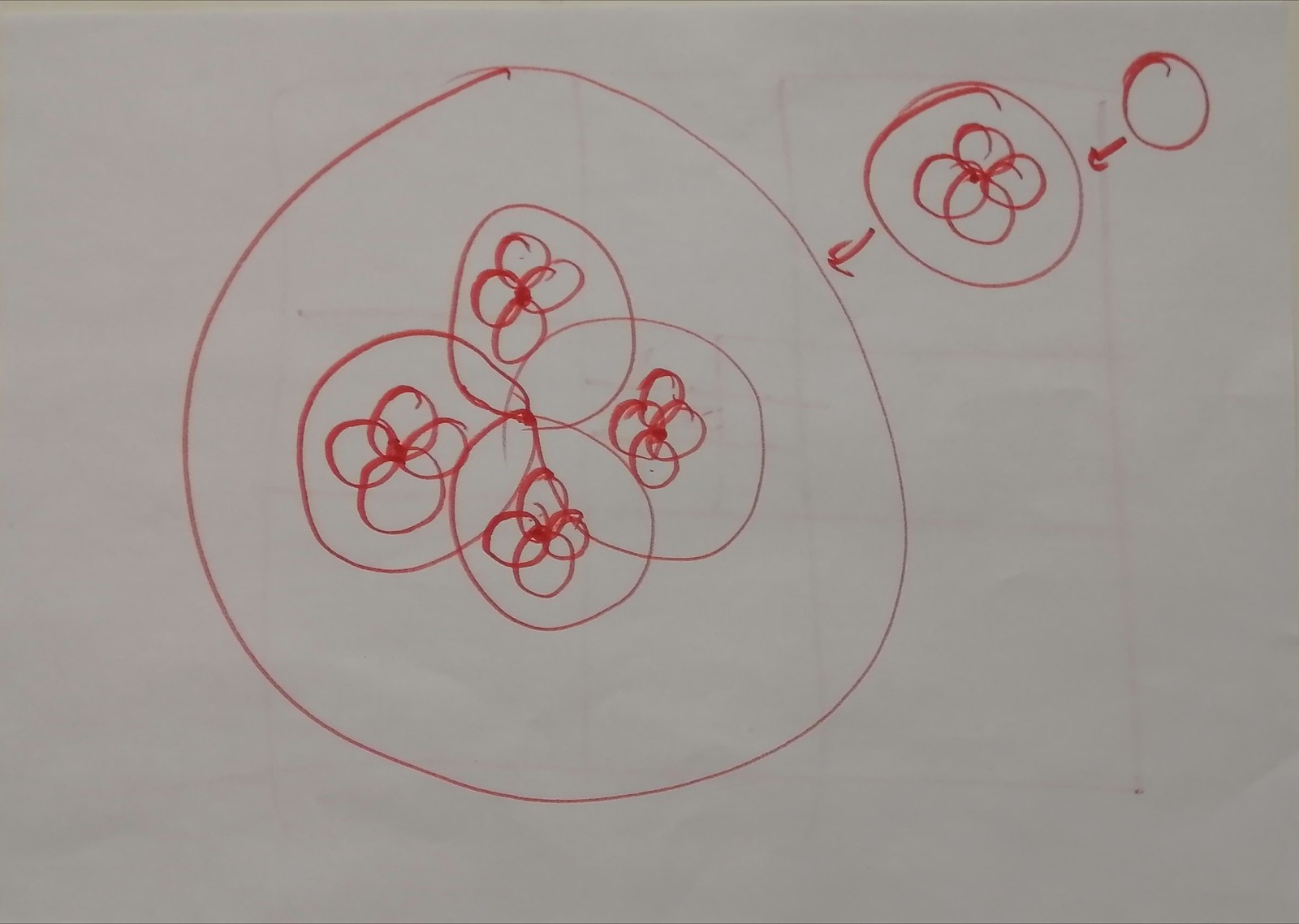This is a detailed, hand-drawn diagram on white paper. At its center, there is a large circle containing four interconnected red rings, overlapping at their centers. Each of these red rings encloses four smaller interconnected red rings, also overlapping at their centers, forming intricate "four-petaled" patterns.

Adjacent to this central motif, in the upper right section, is a single red ring. Inside this ring are four interconnected red rings, similar to the pattern in the larger central circle, overlapping at their centers. Further up and to the right of this motif is another solitary red ring, which is empty in the center.

The composition appears to build progressively outward from the central large circle, illustrating a repeating pattern of interconnected red rings, each layer more complex and nested than the previous.